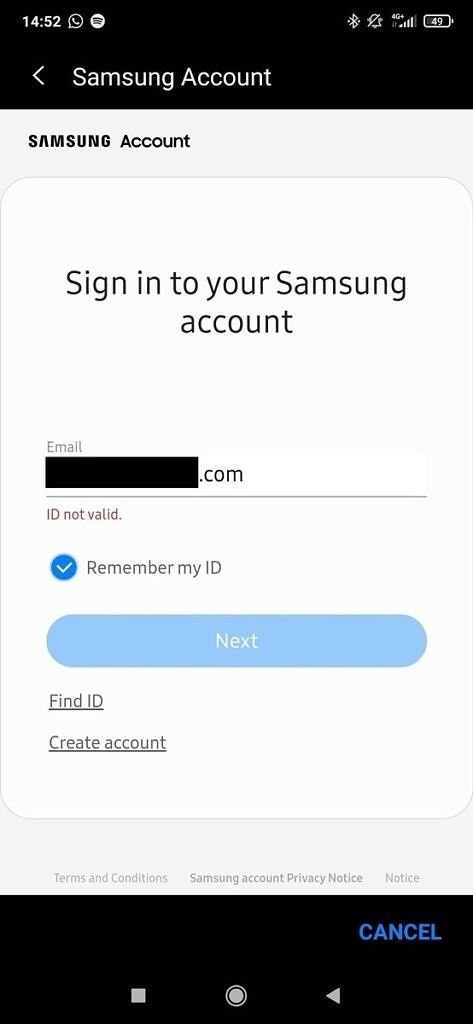The image captures the login screen for a Samsung account on a mobile device. At the top left, there are icons for Bluetooth, a bell (indicating notifications), and a symbol for 4G connectivity. The battery indicator shows 49% remaining. 

Centered on the screen is the text "Sign in to your Samsung account." Below this, there is a text field labeled "Email," accompanied by a black rectangle partially showing a ".com" domain. A horizontal line denotes that the ID entered is not valid, indicated by the text "ID not valid." 

To the right of the email entry field, there is a blue check mark labeled "Remember my ID." Underneath, a light blue oval button displays "Next." Below this button, gray text links are labeled "Find ID" and "Create account."

Further down, there are links to "Terms and Conditions" and "Privacy Notice." At the bottom of the screen, a black bar runs horizontally, containing blue text on the right that says "Cancel." Additionally, there are gray squares in the middle and at the bottom of the interface.

At the very top of the screen, there is another black bar with the title "Samsung account," indicating this is indeed a Samsung account login page.